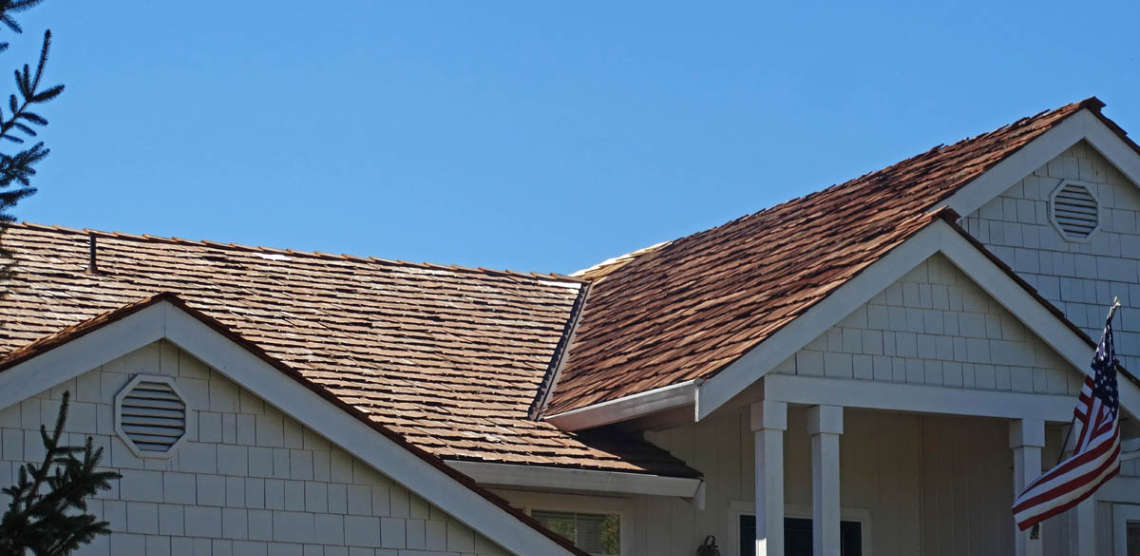This image captures the upper portion of a house, featuring a broad view of its roof and some of the front façade. The house, primarily a light tan or cream color with white outlining, has a shingled brown roof with a clear blue sky as its backdrop, indicating the picture was taken during the day. Prominently, there are two hexagon-shaped vents located near the roof's peak. On the left side of the image, evergreen branches can be seen, hinting at surrounding vegetation. The front of the house showcases two columns, one of which has an American flag mounted on a flagpole, fluttering in the wind. Partial views of a window and a door are visible, although the full extent is obscured. Additionally, a small protrusion that looks like an antenna or a small chimney is noticeable on the roof.